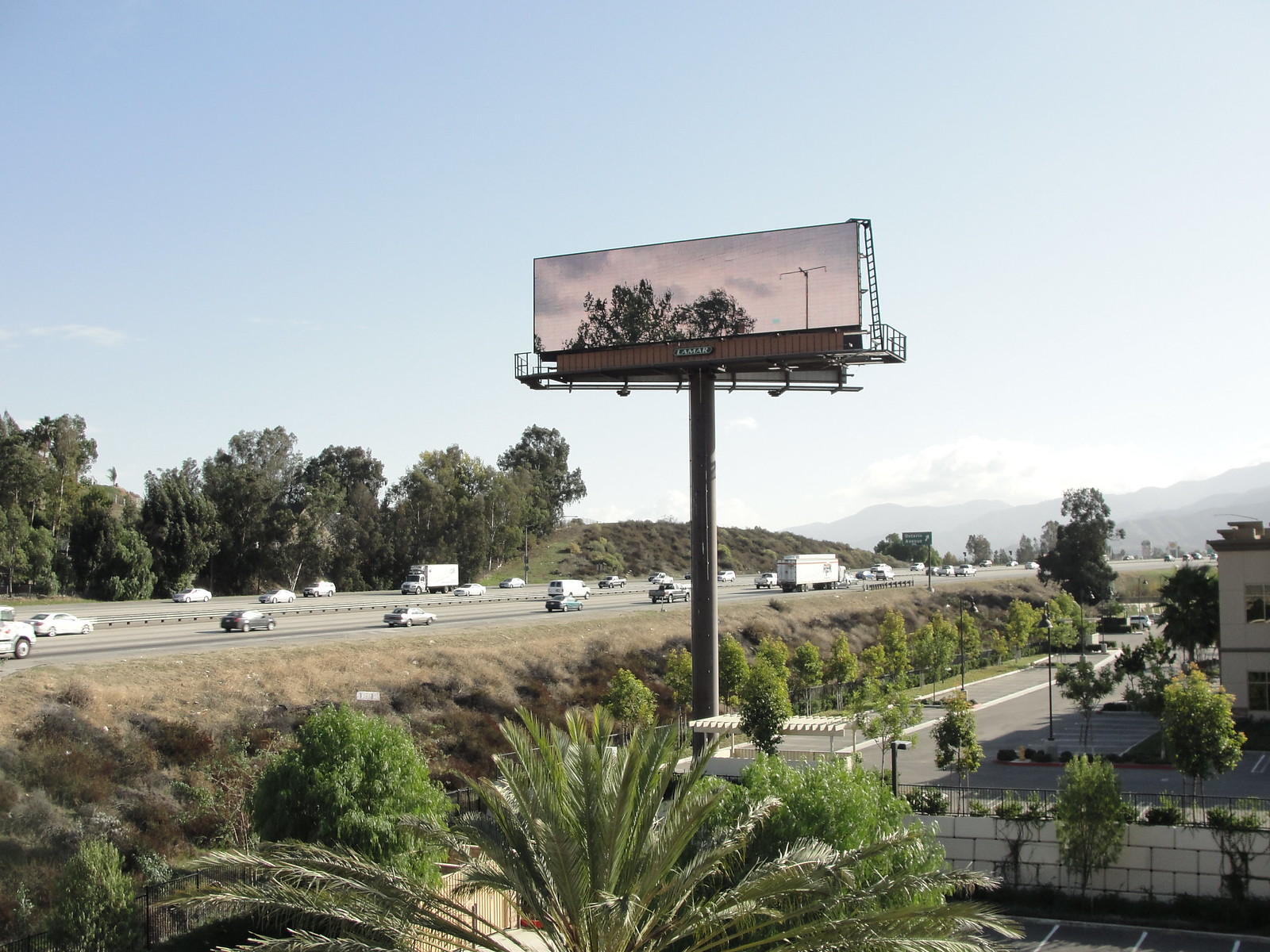A vivid image captures a tranquil landscape where a clear blue sky stretches overhead. In the far distance, the horizon is lined with dark, silhouetted hills. Closer to the foreground, green hills dotted with various bushes and trees emerge, adding a lush vibrancy to the scene. On the left-hand side, a dense cluster of multiple trees stands, contributing to the verdant backdrop.

The foreground features a network of gray streets busy with numerous vehicles, illustrating the pulse of daily life. On the right, amidst the urban sprawl, brush and green foliage intersperse with the asphalt, creating a striking contrast between nature and man-made elements.

There's a notable presence of palm trees, adding an exotic touch to the scenery. A large billboard towers above, prominently displaying images of trees, further emphasizing the thematic fusion of urban infrastructure with natural beauty. The scene is framed with white walls, which, alongside the gray asphalt, provide depth and frame the vivid tableau of contrasting elements.